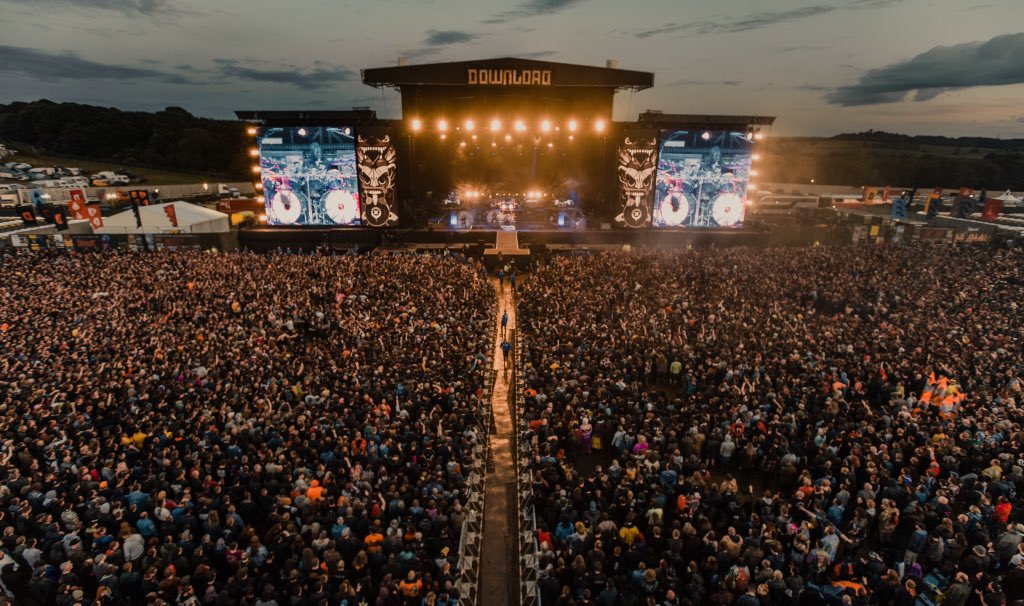The image depicts a grand music concert occurring at dusk, captured from an aerial view in a landscape layout. The center of the composition is dominated by a well-lit stage, prominently displaying the word "Download" at the top. The stage, divided into three sections, is flanked by two large screens on either side, likely projecting live footage of the performance for the vast audience. Above the stage, eight bright lights illuminate the scene, though the performers themselves appear as indistinct figures due to the distance. To the left and right of the stage are sculptures resembling ancient, two-eyed creatures.

Stretching from the stage to the forefront of the image is a clear aisle, facilitating access through the sea of fans that pack the venue, suggesting a highly popular event. The crowd, numbering in the thousands, occupies the bottom half of the picture, appearing as a dense, unbroken mass of enthusiastic concert-goers. Beyond the crowd, the background features a gray, cloud-covered sky with the last light of the setting sun, and a distant mountain range silhouetted against the horizon, indicating the concert’s picturesque, mountainous setting.